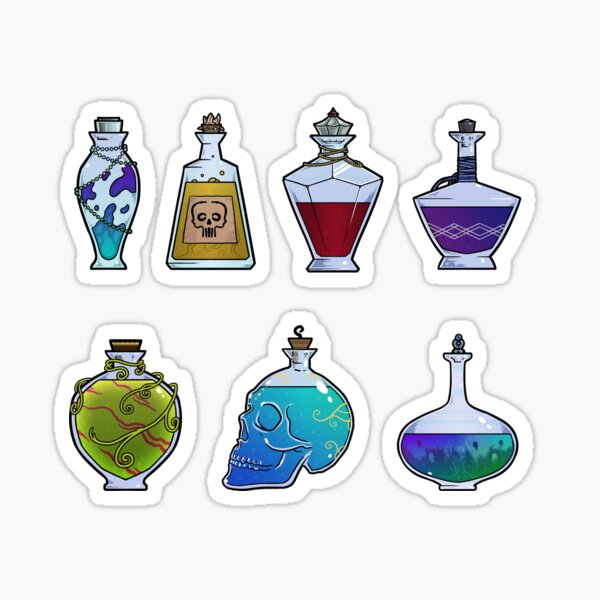This vibrant image showcases seven distinct, computer-generated glass bottles, each featuring various colored liquids and intricate designs. Set against a white backdrop with a light gray border on a lighter gray background, the bottles are meticulously detailed. On the bottom row, the first bottle to the left is heart-shaped, filled with green liquid and sealed with a cork. Next to it is a bottle resembling a skeleton’s skull, viewed from the right profile and filled with blue-green liquid, also corked. The third bottle in this row has a genie-bottle shape, containing bluish-green liquid and topped with a cork.

The upper row starts on the left with a light blue and dark blue bottle adorned with a thin chain wrapped around it and capped with a flat cork. To its right is a tall, tapered bottle holding yellow liquid, featuring a silhouette of a bearded man's head on its front and crowned with a diamond-shaped cork. Following this is a diamond-shaped bottle containing red liquid with a corresponding diamond-shaped cork. Lastly, a bottle with an octagonal shape houses purple liquid and is sealed with a cork.

Among these diverse designs, some bottles are angular, while others are elegantly curved, each contributing to the overall intricate and imaginative scene.